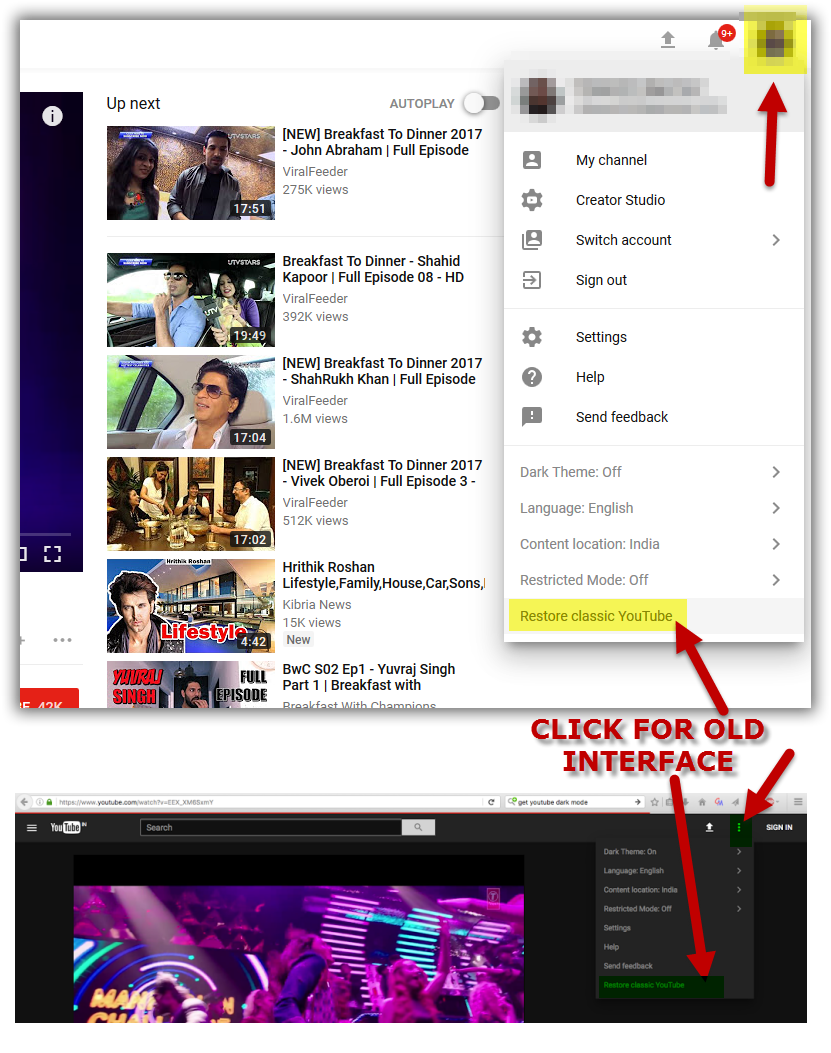A blurred image highlights a creator's studio interface showcasing various video titles. At the top, a directory labeled "Up Next" features an autoplay button option. To the right, a menu lists several options including "My Channel," "Creator Studio," "Switch Account," "Sign Out," "Settings," "Help," "Send Feedback," along with toggles for "Dark Theme (On/Off)," "Language: English," "Content: Location - India," "Restricted Mode: Off," and "Restore Classic YouTube."

On the left side, detailed video titles and thumbnails are visible:
1. "Breakfast to Dinner 2017, John Abraham Full Episode," posted by Viral Feeder, with 276,000 views. The video is 17 minutes and 51 seconds long, featuring a man and a woman.
2. "Breakfast to Dinner, Shahid Kapoor Full Episode," posted by Viral Feeder, with 392,000 views. This 19-minute and 49-second video shows a man and a woman sitting in the backseat of a car.
3. "Breakfast to Dinner 2017, Shakira Khan Full Episode," also by Viral Feeder, with a substantial 1.6 million views. The episode lasts 17 minutes and 4 seconds and features a man in a car wearing sunglasses, a white shirt, and a tan jacket.
4. A new entry titled "Breakfast to Dinner 2017, Vivek Oberoi Full Episode 3," from Viral Feeder, accumulating 512,000 views. This 17-minute and 2-second episode shows three people seated at a table.
5. Finally, a different segment under the title "Lifestyle: Hrithik Roshan Lifestyle Family House Car Sons," from Qubria News, with 1.5 thousand views, lasting 4 minutes and 42 seconds.